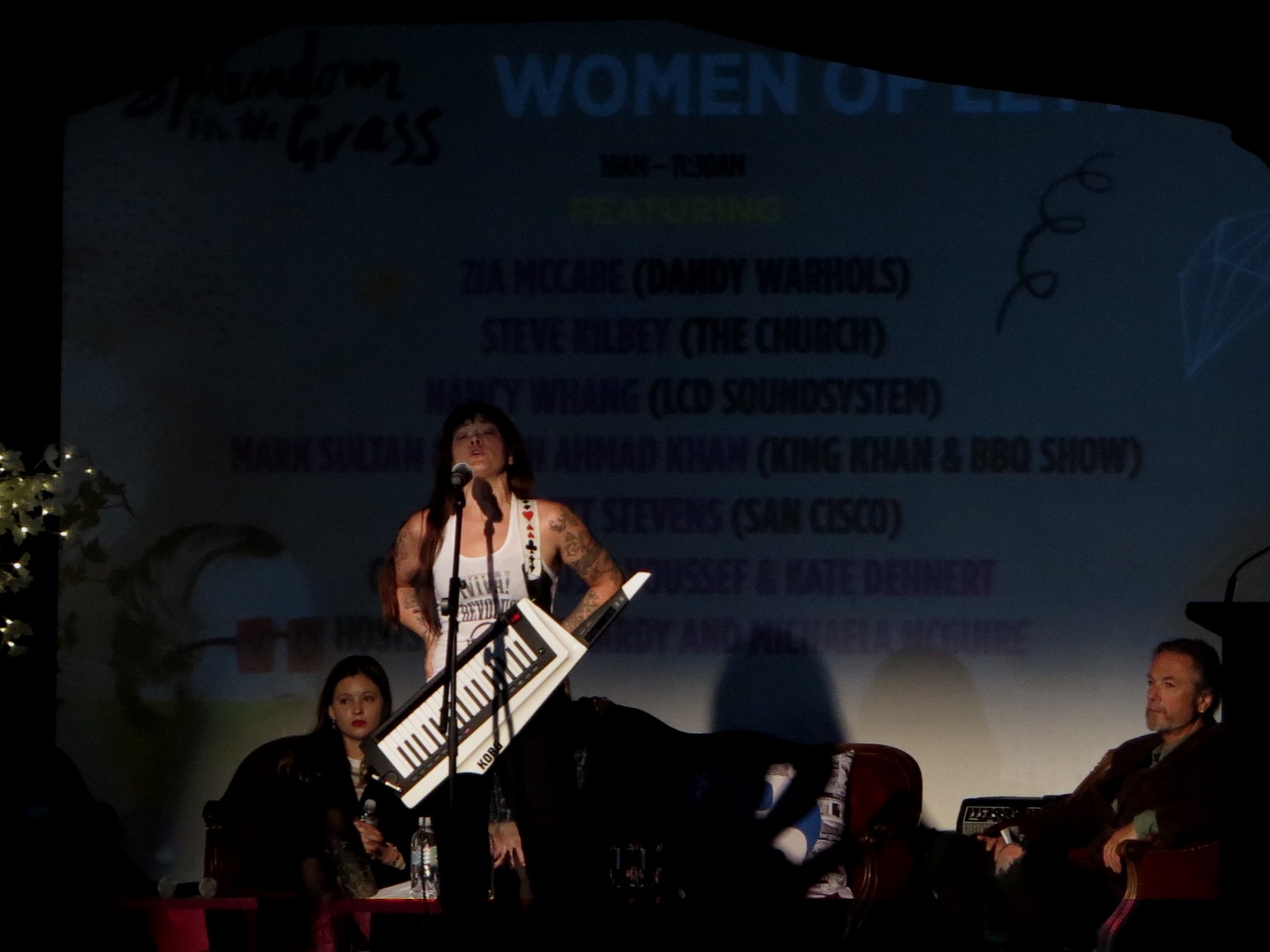The image captures a dimly lit stage, likely inside a room, where a woman stands illuminated by a spotlight. She has long black hair and tattoos covering her arms, embodying a commanding presence as she performs with a keytar, the black and white keys of the instrument distinct under the light. She is wearing a white muscle shirt that reads "Viva Revolution". Her mouth is open, and her eyes are closed, suggesting she is deeply engaged in her performance, with a black microphone on a stand in front of her.

Behind her is a projection screen displaying the words "Women of" at the top, followed by a list of names and phrases, one of which is "featuring Zia McCabe". The other details on the screen are hard to make out due to the lighting. On stage with her, two people sit on chairs further back: a woman with pink or red lipstick looking off to the side, and an older man on the bottom right, both part of the scene but not the main focus. To the left of the central action, there is what seems to be part of a tree or leaves, and a blue and white pillow is visible on a sofa behind the performer. The ambiance is a blend of white, brown, and hints of purple, adding to the atmosphere of an intimate live performance. Shadows, including that of the performer, play upon the white wall, completing the evocative scene.